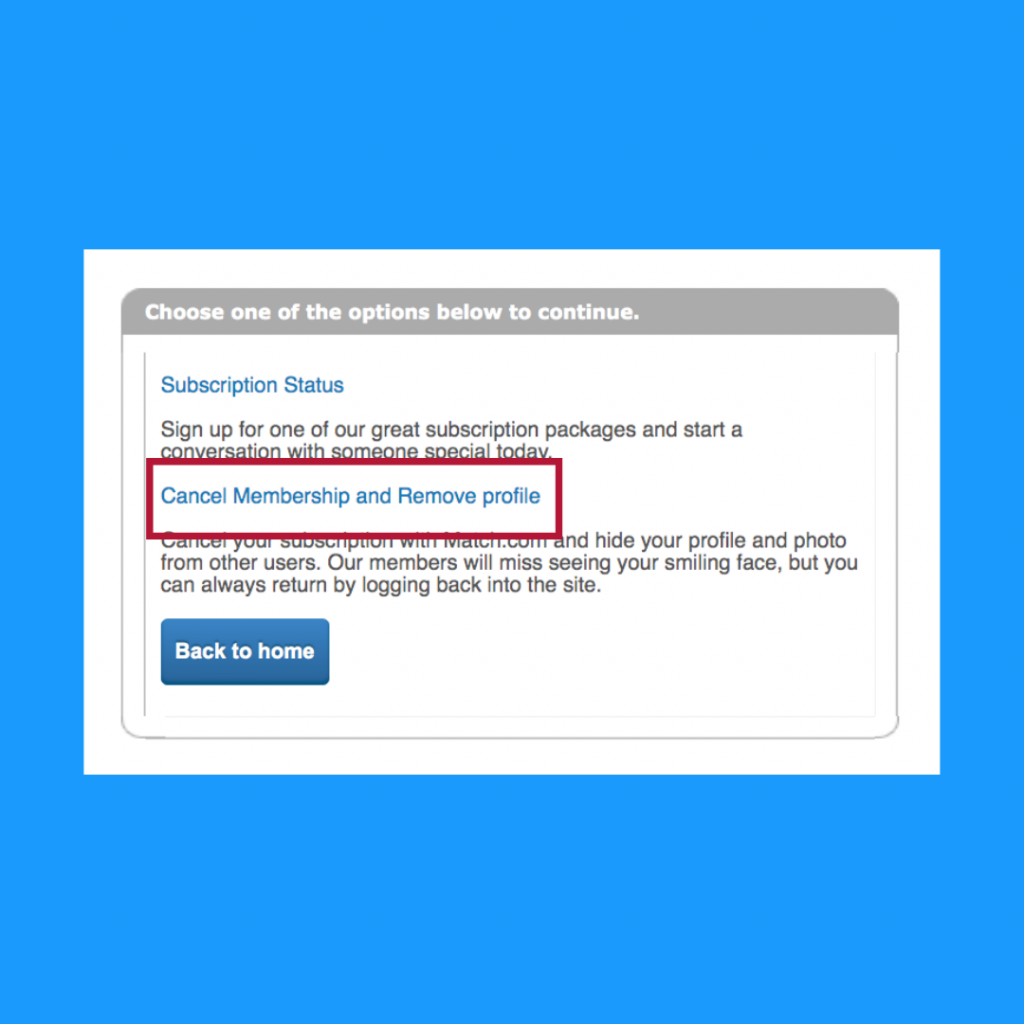The image features a sleek user interface on Match.com's platform, set against a blue background with a white rectangular box in the center. Within this box, users are prompted to choose between two options. 

The first option, titled "Subscription Status," encourages users to "sign up for one of our great subscription packages and start a conversation with someone special today," suggesting the nature of the dating app. The second option, "Cancel Membership and Remove Profile," allows users to cancel their subscription with Match.com and hide their profile and photo from other members. It reassures users that while other members will miss seeing their smiling face, they can always return by logging back in.

Additionally, there's a "Back to Home" button for users who decide not to make any changes. This button is blue with white font, aligning with the platform's color scheme. All action links are in blue, while the regular text is in black, ensuring clarity and ease of navigation.